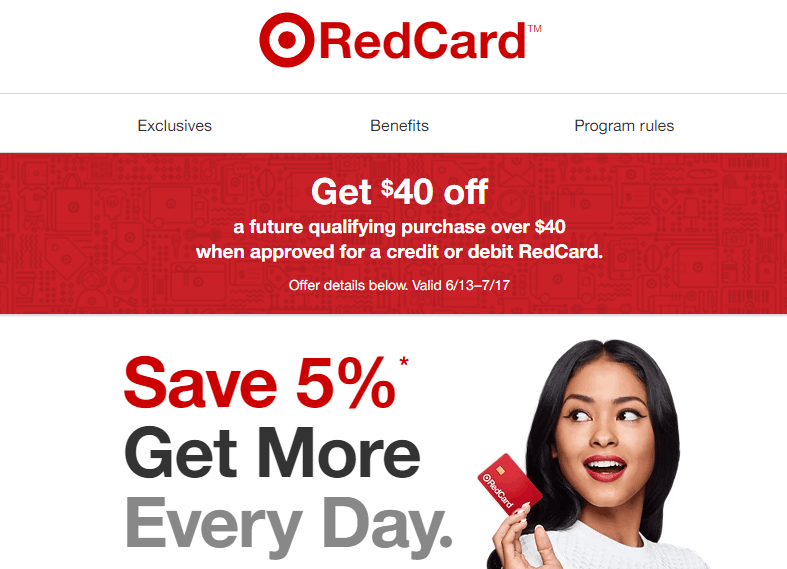**Target RedCard Promotional Ad**

The image depicts a promotional ad for Target's RedCard, resembling a typical webpage from the Target website. The background is primarily white, featuring a mixture of red and black text. At the top, the iconic red Target bullseye logo is prominently displayed next to the phrase "RedCard" written in red. Below this, a thin gray line separates the header from the main section, which includes three clickable options: "Exclusives," "Benefits," and "Program Rules."

A large red rectangle spans the width of the image, containing a special offer in white text: "Get $40 off a future qualifying purchase over $40 when approved for a credit or debit RedCard. Offer details below. Valid 6/13 to 7/17." The red rectangle's background is adorned with subtle, light-gray illustrations of various shopping-related items, including tags, clocks, and lamps, contributing to a shopping theme.

Below the red rectangle, bold red text announces "Save 5%," followed by "Get more" in black, and "every day." in gray. 

To the right of this text, an image of a joyful Asian woman with black hair and red lipstick is displayed. She is holding up a RedCard in her right hand, her mouth open in an expression of surprise and happiness, and she is looking towards the left side of the image. 

The entire layout and design elements effectively convey the benefits and excitement associated with the Target RedCard.